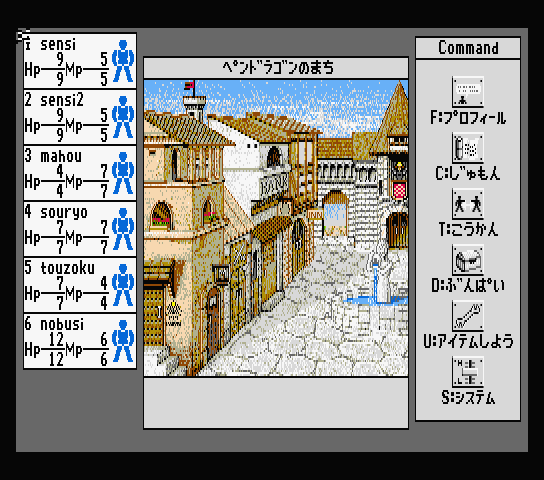The image appears to be a screenshot from a vintage computer game, likely from the early eras of pixel art and low-resolution graphics. At the center of the image is a cobblestone courtyard, highlighted by a fountain featuring a female figure holding an object, from which water is cascading into the blue basin below. The courtyard is encircled by medieval-style buildings, with distinct signs and banners indicating places such as a "bank" and an "inn." A castle turret adorned with a red flag is also visible, contributing to the overall medieval ambiance.

Above these buildings, there are inscriptions in Asian script. The image is noticeably pixelated, reinforcing its retro aesthetic. 

On the left side of the image, there is a pixelated avatar of a blue figure standing with feet apart, repeated six times. Accompanying this avatar are the details "Sensai, HP: 9/9, MP: 5/5," suggesting a character's health and magic points common in role-playing games (RPGs).

On the right side, the word "Command" is prominently displayed, followed by six clickable gray boxes, each featuring symbols or icons that likely represent different possible actions or commands in the game. While the exact nature of the symbols is unclear, they contribute to the interactive elements typical of RPG interfaces.